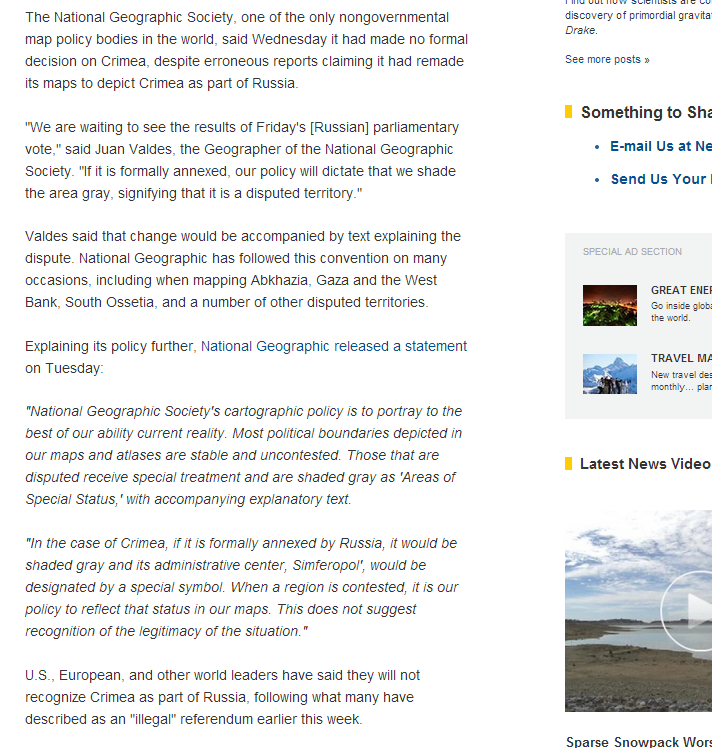This image depicts a page layout that appears to be from either a website or a magazine, predominantly filled with text. On the left-hand side, there are six to seven paragraphs of black text. The first paragraph announces that the National Geographic Society, known as one of the few authoritative bodies on map policy, issued a statement on Wednesday. It clarified that no definitive decision had been made regarding the depiction of Crimea on its maps, despite incorrect reports suggesting otherwise. Further down, there are several quotes presented, including one notable extract which clarifies that if Crimea were officially annexed by Russia, it would be shaded gray on the map, and its administrative center, Simferopol, would be marked by a special symbol. It is emphasized that while a region's contested status is depicted on maps, this does not imply any recognition of the situation's legitimacy.

On the right-hand side of the layout, there is a narrower vertical column featuring additional textual content and several images. At the top, a section titled "Something to Share" includes an email hyperlink and a "Send Us Your Something" hyperlink, both highlighted in blue, with a small gray box underneath. Below, a special ad section is present, comprising two square images accompanied by some text to their right. Further down, there is a "Latest News Video" section that displays a video playlist. The thumbnail image shows a marshy landscape adjacent to a sandy or dirt area with a small body of water and the sky above. The label beneath this thumbnail reads, "Far Snowpack."